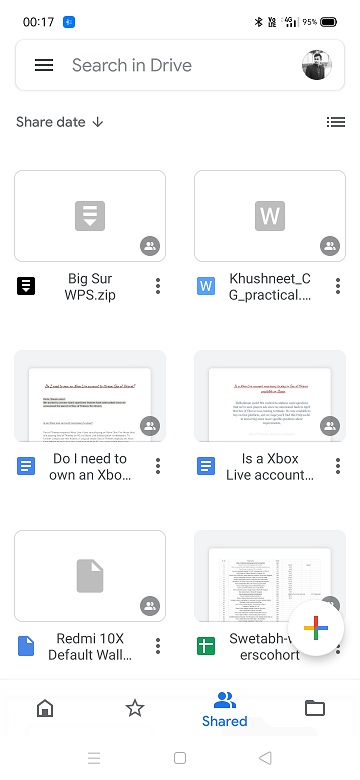**Detailed Caption:**
Displayed on a smartphone screen under the "Websites" category, the interface is active and showcasing various document listings and status indicators. At the very top, there is a status bar displaying "Bluetooth is enabled" and the battery level at "95%." Directly beneath, a white bar edged in light grey features a menu icon, represented by three horizontal bars.

Central to the display is a black-and-white photograph of a man wearing a suit. Below this image, the text reads "Share Date" accompanied by a downward-pointing arrow, suggesting the option to view or modify sharing settings. The next listed item is a file named "Big Sur WPS.zip," which is followed by an icon of three vertical dots indicating additional options. Next to this file is another titled "Cushneet CG Practical," which is identified with a 'W' icon signifying a Word document.

Further down, the screen lists additional documents: "Do I need to own an Xbox?" and "Xbox Live Account," both recognized with Word document icons. At the bottom of the screen, it concludes with the statement "This is shared," indicating that the contents are accessible to others.